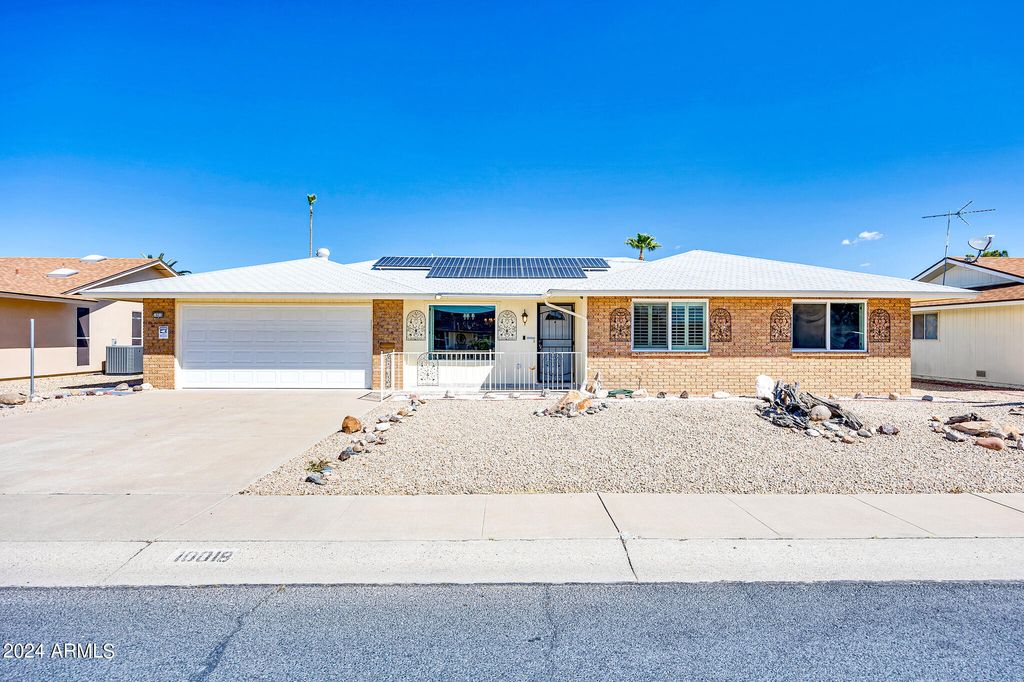This vibrant photograph captures a sunlit suburban street showcasing a contemporary, single-story ranch-style home, distinguished by its light brick exterior with white trim and a white roof. The address 10018 is painted on the curb in front of the well-maintained sidewalk. The property is part of a larger housing development evident from similar houses in the background. Dominating the simple, gravel-covered yard accented with decorative stones and timbers is a long driveway leading to an attached two-car garage. The house features solar panels centrally placed on the roof, indicative of modern energy-efficient design. The facade includes two sets of double windows to the right of a secured front door, which boasts a half-moon window with a peephole and protective bars. The entrance is highlighted by a small railing and decorative arches, possibly shutters, adding a quaint charm. Behind the homely structure, under a bright blue sky, a small tree peeks into the scene, completing this picturesque suburban snapshot from a 2024 ARMLS real estate listing.